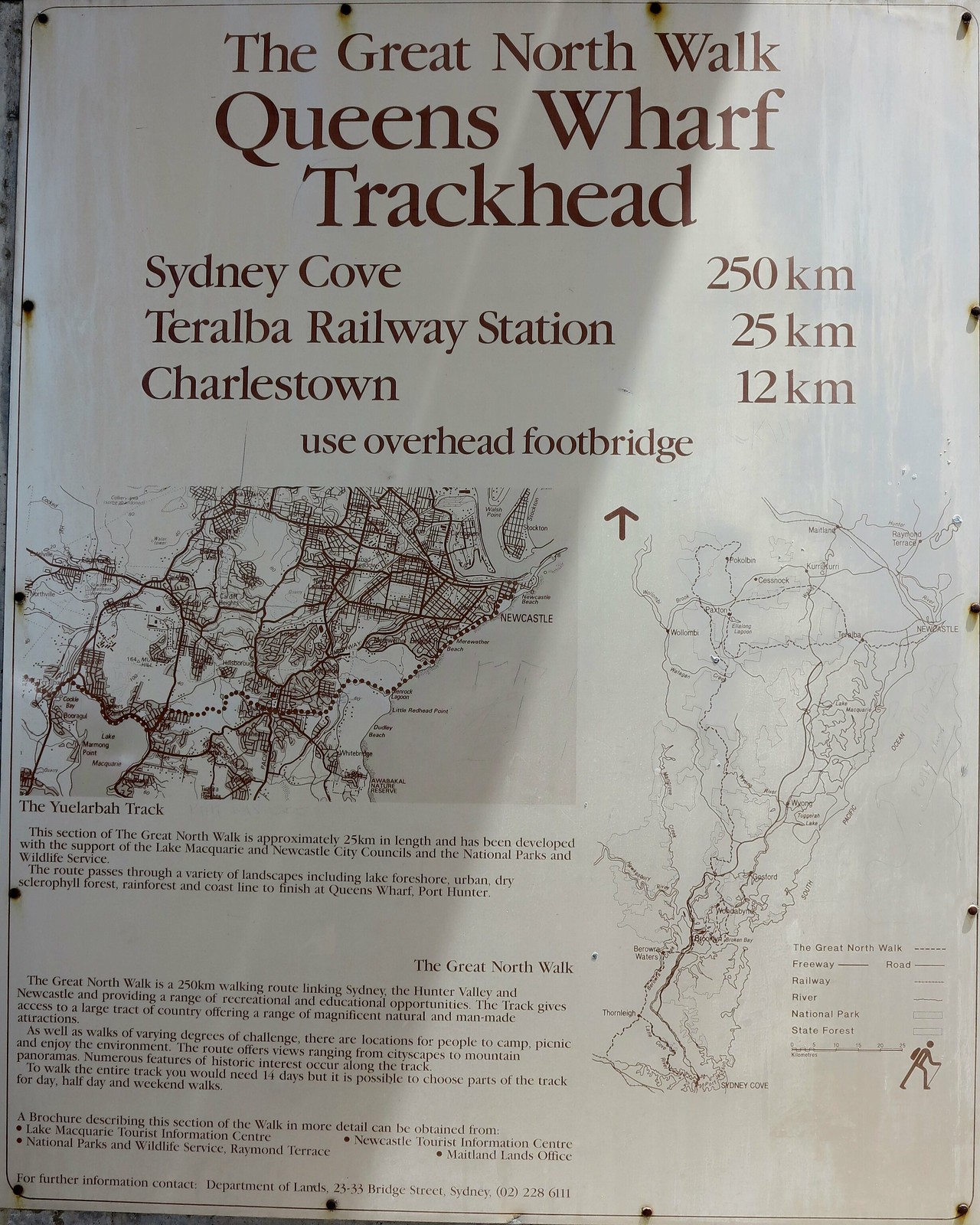The image is a photograph of an information board mounted on a white background, secured by screws at its corners. The poster prominently displays the title "The Great North Walk" at the top in black text. Below the title, it lists key locations and distances: "Queens Wharf Trackhead," "Sydney Cove, 250 km," "Toralba Railway Station, 25 km," "Charlestown, 12 km," and "Hughes Overhead Footbridge." On the right side of the poster is a detailed map of a peninsula illustrating walking trails, while the left side features a simpler, general city map that includes Newcastle, showing roads and areas. The board also contains two unreadable paragraphs. The first, located under the heading "Y-U-C-L-A-R-B-A-H Track," and the second detailed paragraph underneath the title "The Great North Walk." The entire poster is monochromatic with black text on a white background.